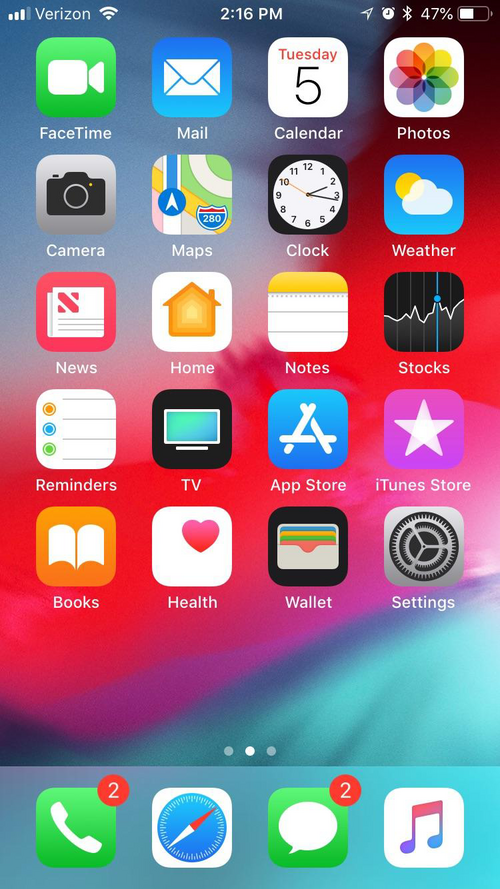This image captures the home screen of a smartphone. Detailed information visible includes:

- **Top Bar:** 
  - Time: `2:16 PM`
  - Signal strength indicator
  - Service provider: `Verizon`
  - Wi-Fi signal icon
  - Battery percentage at `47%`
  - Additional icons for Bluetooth, alarm, and messages visible on the right.

- **Wallpaper:** 
  - The background features a mix of vibrant colors including blue, red, green, and some purple shades.

- **App Icons:**
  - **First Time:** Green and white icon
  - **Mail:** Blue and white icon
  - **Calendar:** Shows the date `Tuesday 5`
  - **Photos:** Multicolored flower-like shape on a white background
  - **Camera:** Black camera icon
  - **Maps:** Grey background with a map icon
  - **Clock:** White clock on a black background
  - **Weather:** Blue background with a white cloud and a yellow sun
  - **News:** Red background with a newspaper icon
  - **Home:** Yellow house on a white background
  - **Notes:** White and yellow icon
  - **Stocks:** Graph icon in black, white, and blue
  - **Reminders:** Notes-like icon
  - **TV:** Blue TV on a black background
  - **App Store:** Blue and white icon
  - **iTunes Store:** Purple background with a white star
  - **Books:** Orange background with a white book
  - **Health:** White background with a red heart
  - **Wallet:** Black icon with a wallet containing blue, yellow, green, and pink cards
  - **Settings:** Grey icon with black gears

- **Dock:**
  - **Phone:** Green icon with a white call symbol, having a red badge indicating `2` notifications
  - **Safari:** Blue icon with a red and white compass needle
  - **Messages:** Green icon with a white text bubble, also with a red badge displaying `2` new messages
  - **Music:** White icon with a red music note

The arrangement showcases a well-organized and visually appealing interface with various essential apps for daily use.